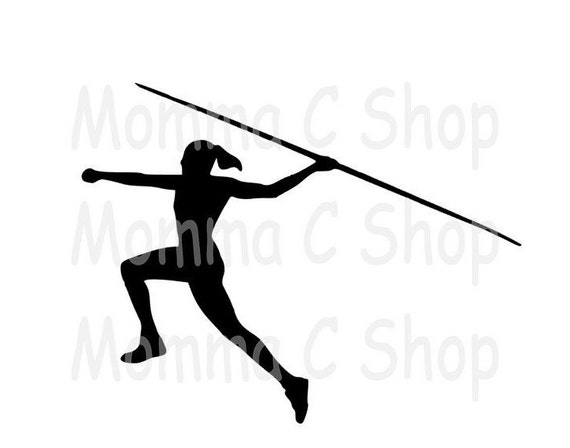The image is a graphic design representation of a woman depicted in a dynamic, mid-leap pose. She is entirely in black silhouette, facing left, with her left leg raised in front of her and her right leg trailing behind. The woman appears to have a ponytail, suggested by the hair extending from the back of her head. Her right arm is fully outstretched in front of her, with her hand in a fist, while her left arm is holding a long spear or javelin, pointed at both ends. The length of the spear spans from the top to the right edge of the image, larger than the figure herself. The figure appears to be in a powerful stance, as if preparing to throw the javelin. Overlaying the entire image are three translucent, light gray watermarks that read "MOMMACSHOP," with each letter capitalized and repeated across the image. The branding slightly obscures but does not dominate the detailed silhouette artwork.